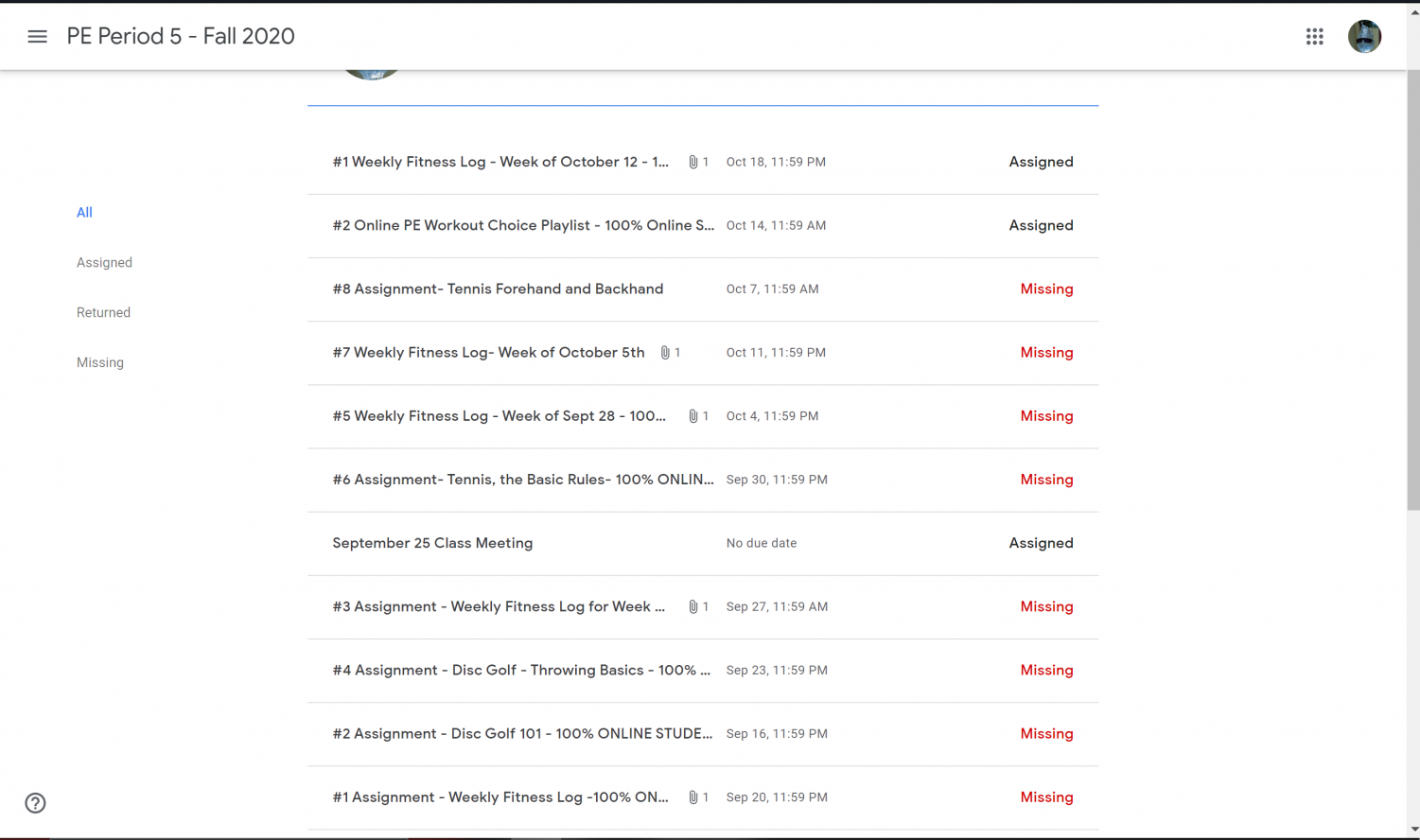The image depicts a page with a primarily white background adorned with a mix of black and red text. In the top left corner, three horizontal lines symbolize a settings menu or dropdown window. Next to it, on the far right, there is an identifier "PE.5-Fall2020" and an icon comprising a square made up of dots.

Centrally located on the page is a detailed list of assignments related to an online Physical Education (PE) class. The list includes:

1. **Weekly Fitness Log**: Week of October 12th (assigned)
2. **Online PE Workout Choice Playlists**: Fully online (assigned)
3. **Assignment Tennis – Forehand and Backhand**: Not yet completed (assigned)
4. **Weekly Fitness Log**: Week of October 5th (missing)
5. **Weekly Fitness Log**: Week of September 28th (missing)
6. **Assignment Tennis – Basic Rules**: Fully online (missing)
7. **September 25th Class Meeting**: No due date (missing)
8. **Weekly Fitness Log**: Week of missing assignment (missing)
9. **Disc Golf – Throwing Basics**: Fully online (missing)
10. **Disc Golf 101**: Fully online (missing)
11. **Weekly Fitness Log**: Fully online (missing)

On the left sidebar, there is a navigation section with options labeled "All," "Assigned," "Returned," and "Missing," with the "All" category currently highlighted.